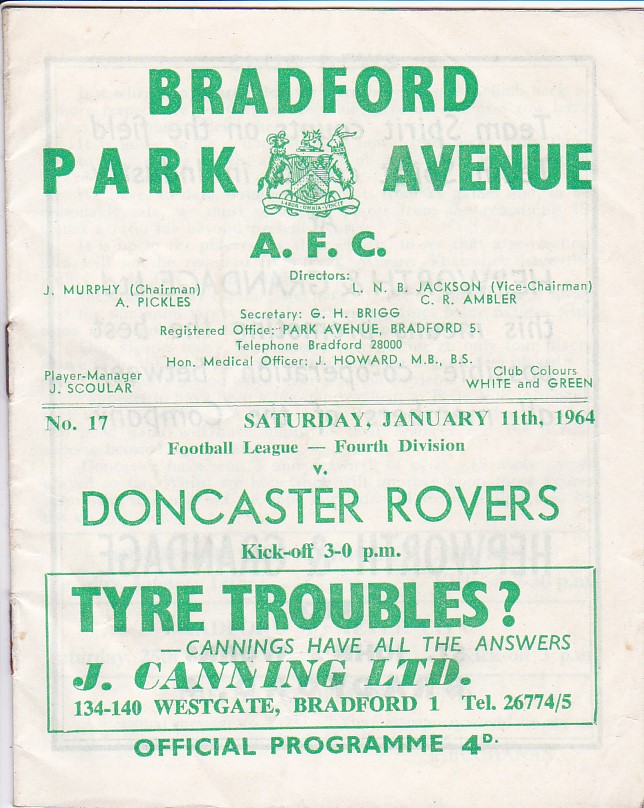This image is of a page from a vintage football program dated Saturday, January 11, 1964, for a match in the 4th Division of the Football League between Bradford Park Avenue and Doncaster Rovers, with a kickoff at 3 p.m. The back of the page has an aged white cream color, and all the text is printed in green. Along the top, it prominently reads "Bradford Park Avenue AFC." Between "Park" and "Avenue," there is a small but detailed logo featuring a shield held up by two or three indistinct animals. 

Below this header, the text lists the club's key officials: Jay Murray as Chairman, L.N.B. Jackson as Vice Chairman, A. Pickles and C.R. Ambler as Directors, and G.H. Brigg as Secretary, with the registered office located at Park Avenue, Bradford 5, and a telephone number of Bradford 28000. The Medical Officer is listed as J. Howard, M.B.B.S., and J. Skolar is the Player Manager. The club colors are noted as White and Green.

Further down, the program is marked as Number 17. An advertisement is placed within an outlined rectangle at the bottom of the page, reading: "Tire Troubles? Cannings have all the answers. Jay Cannings, Ltd. 134-140 Westgate, Bradford 1. TEL 26774-5." The page is identified as the "Official Program," priced at 4D.